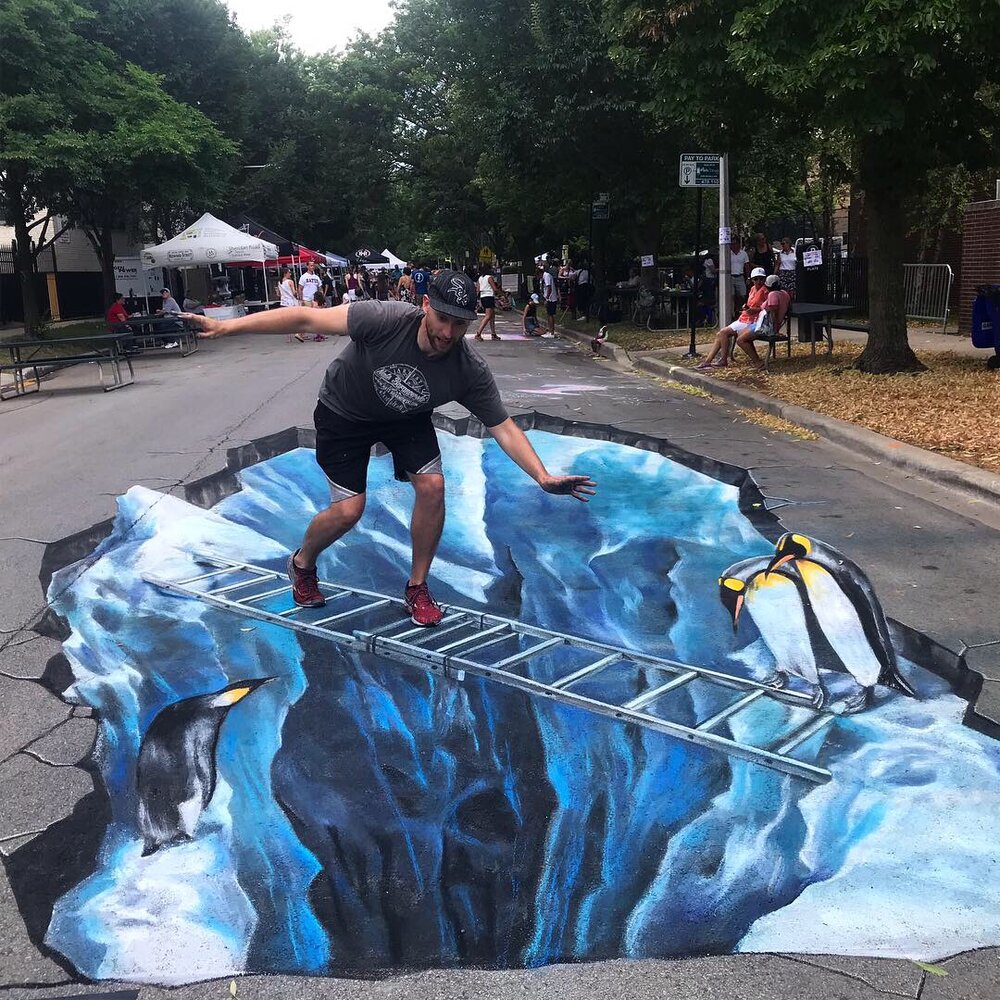This full-color daytime photograph, taken outdoors with natural light, captures a fascinating optical illusion painted onto a city street. The square image, framed by a canopy of tree leaves at the top, shows a busy scene with people milling around and various white tents and booths set up in the background. Central to the photo is an expertly drawn optical illusion, making it appear as though the concrete street has a giant crevice filled with icy depths. A painted ladder stretches across this faux abyss, reaching from the snowy edges on the upper left to the lower right of the crevice. 

Positioned on this illusionary ladder are painted penguins looking down into the crevice, enhancing the artwork's realism. Adding to the effect, a real man, dressed in a black hat, a gray shirt with a white design, black shorts, and red tennis shoes, pretends to walk across the ladder, striking a balancing pose with his arms extended to either side. This dynamic interaction blurs the lines between reality and art.

To the right, the street curb and a bench with a couple of people seated next to a road sign are visible. The ground is scattered with either dead leaves or wood chips, adding texture to the scene. The image beautifully captures the blend of street art and urban life, with the distant view showcasing various people walking normally along the street lined with trees.